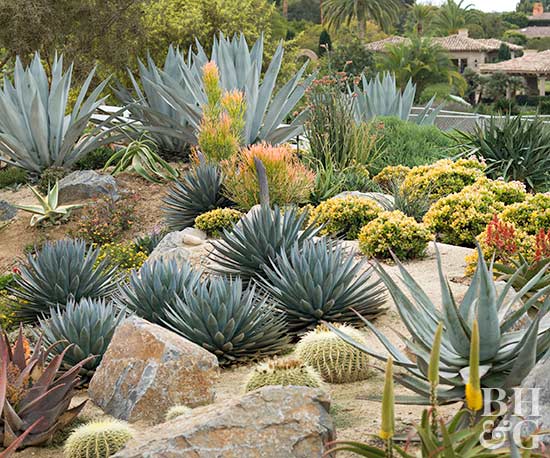The photograph, taken on an overcast day, features a rocky, desert landscape interspersed with several types of succulents and cacti, thriving amidst the rugged terrain. Large rocks and mini boulders punctuate the scene, nestled between small hills of dirt and soil. The greenery includes succulents of various sizes and shapes, predominantly in dull and light greens, some forming ball-like clusters with spiky leaves, and others shorter and rounder resembling barrel cactus. Notably, there are yellow spiked ball cacti and purple spiky plants adding visual interest. Small desert shrubs, some yellow and others green and orange, are scattered throughout. In the distance, white and tan houses are visible, providing a contrast to the natural setting. Additionally, the bottom right corner of the photograph features the letters B, H, and G in white light font.